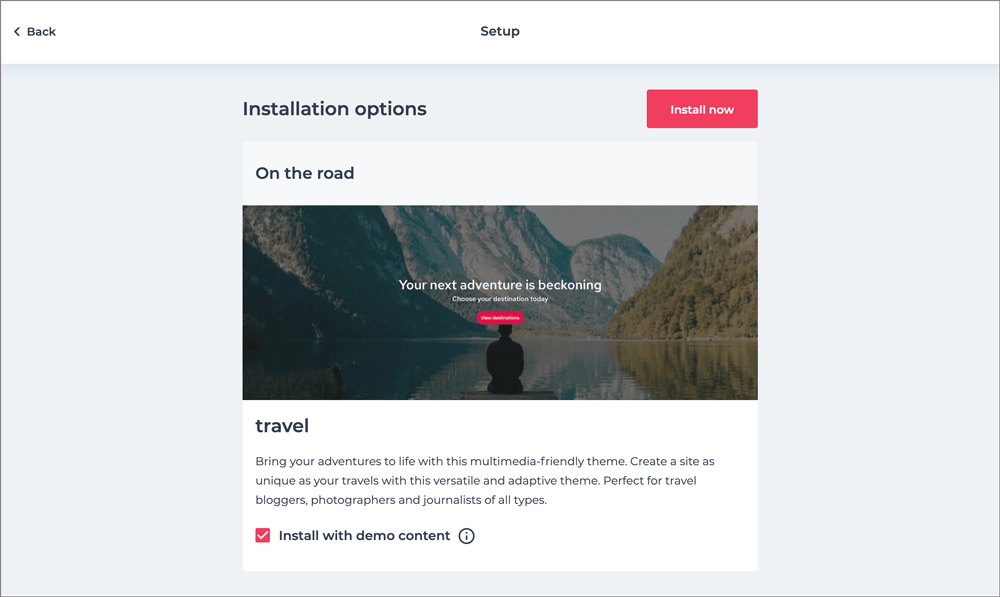The screenshot captures a website interface with a clean and organized design. The top section features a solid white background with a left-facing arrow and the word "Back" (with a capital 'B') written next to it on the left side. Centered at the top is the word "Setup" with a capital 'S'.

Below the top section, the background shifts to a light-to-medium gray shade with the heading "Installation Options" prominently displayed in bold text and a capital 'I'. Adjacent to this heading is a red button labeled "Install Now" in white text.

Continuing down the page, the background lightens to a lighter gray. This section is headed by a banner with the phrase "On the Road" where the 'O' is capitalized. Beneath this banner is an image depicting a landscape with two mountains, one on the left and one on the right, the latter featuring more trees. A waterway runs between the mountains, and a silhouette of a person (indistinguishable gender) is visible from behind, standing in a dark hue.

Embedded within the image is white text that reads, "Your next adventure is beckoning. Choose your destination today." Additionally, there is a small red tab with some illegible white text.

Below this image, there is a white banner containing the word "Travel" and a subheading "About Travel." Directly underneath this banner is a red square featuring a white checkmark and the inscription "Install with Demo Content."